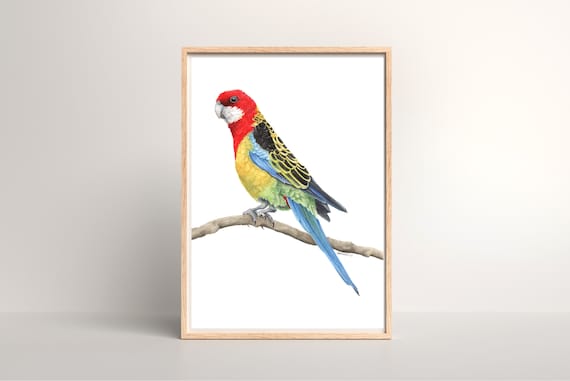This is a detailed photograph of a framed piece of art depicting a colorful parrot perched on a tree branch. The frame of the artwork is wooden, lending a rustic touch to the piece. The picture is leaning against a gray wall, with a darker gray surface beneath it. The background within the artwork is white, allowing the vibrant colors of the parrot to stand out prominently. 

The parrot itself is the focal point of the artwork, with its body turned to the left while its head faces forward. Its head is a striking red color, complemented by a white beak and a beady black eye. The bird's chest is yellow, and its feathers boast a mix of blue, black, gold, and green hues. The wings have baby blue and dark blue feathers extending to a long blue tail feather. The scene captures the parrot in a roosting position, centered within the frame. This indoor setting provides no textual distractions, focusing entirely on the vivid depiction of the bird. The medium of the artwork might be an artistic drawing, painting, or digital print, showcasing the parrot with meticulous attention to detail and color.